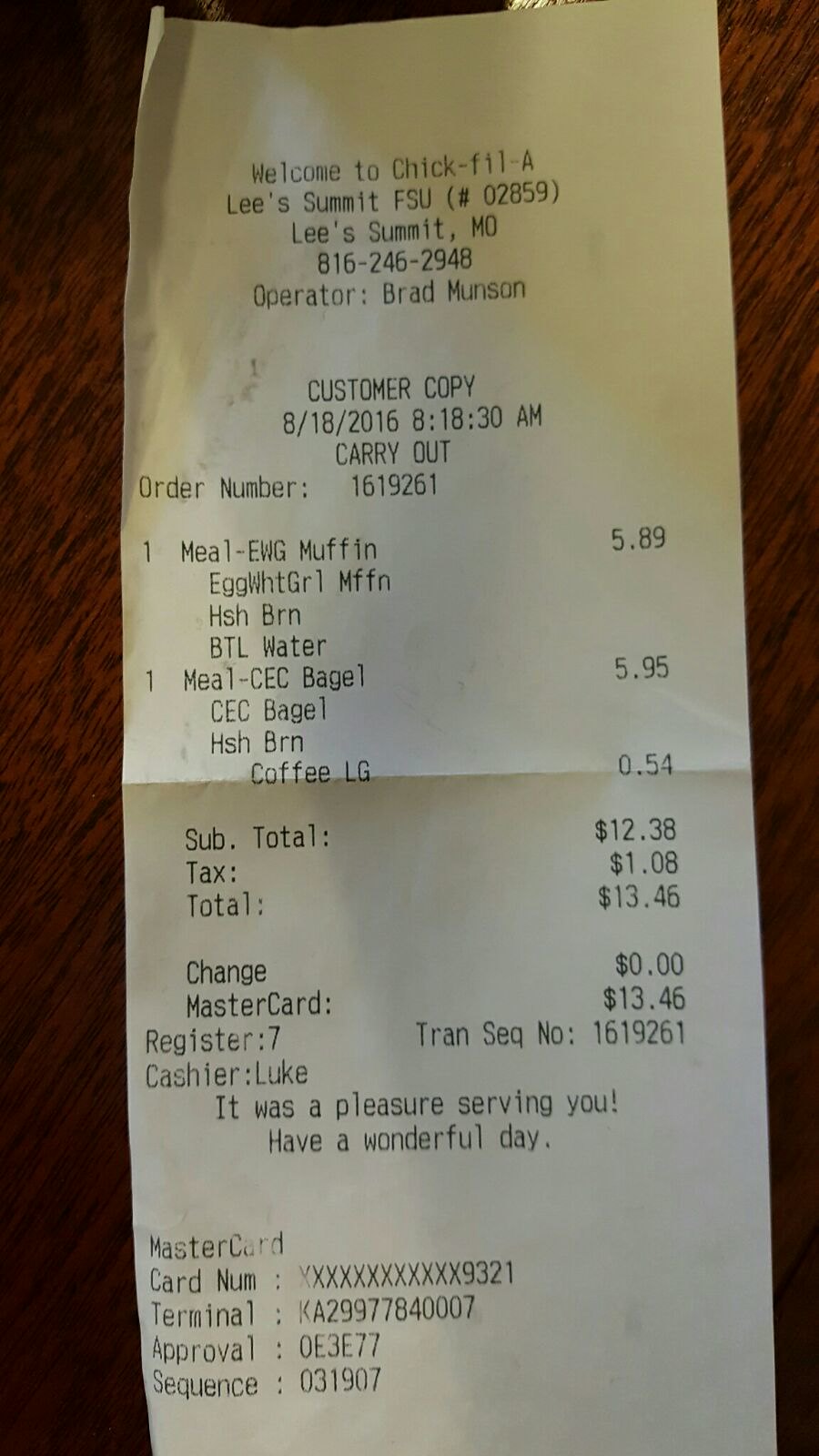A Chick-fil-A receipt is displayed on a dark wood grain background. The receipt header reads "Welcome to Chick-fil-A Lee's Summit FSU" in Lee's Summit, Missouri, along with the contact number, 816-246-2948, and the operator's name, Brad Munson. This customer copy, paid with a MasterCard, lists the cashier as Luke. The receipt concludes with a friendly message: "It was a pleasure serving you. Have a wonderful day." The order includes an English muffin with egg white, hash browns, and water, as well as a bagel with hash browns and coffee. The total amount of the purchase is $13.46.